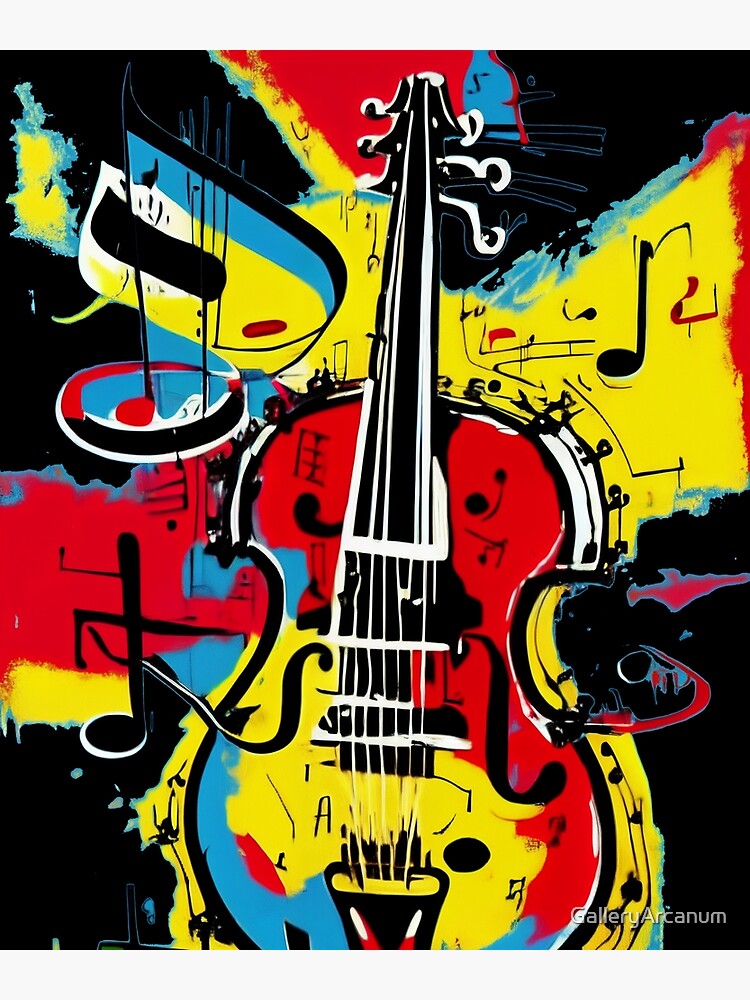This image features a vibrant and dynamic artwork, likely created digitally but reminiscent of traditional paint techniques. At its center, a stringed instrument, resembling a bass or cello, commands attention with its bold outline in black and white. The cello bursts with intense hues of red, yellow, and blue, bringing life and energy to the piece. Its white strings add a stark contrast, enhancing the visual complexity. The background is a deep, immersive black, while dramatic swathes of red and yellow sweep across the composition, creating a sense of movement and excitement. Scattered musical notes further contribute to the chaotic, abstract nature of the artwork, suggesting a symphony of creativity and expression.